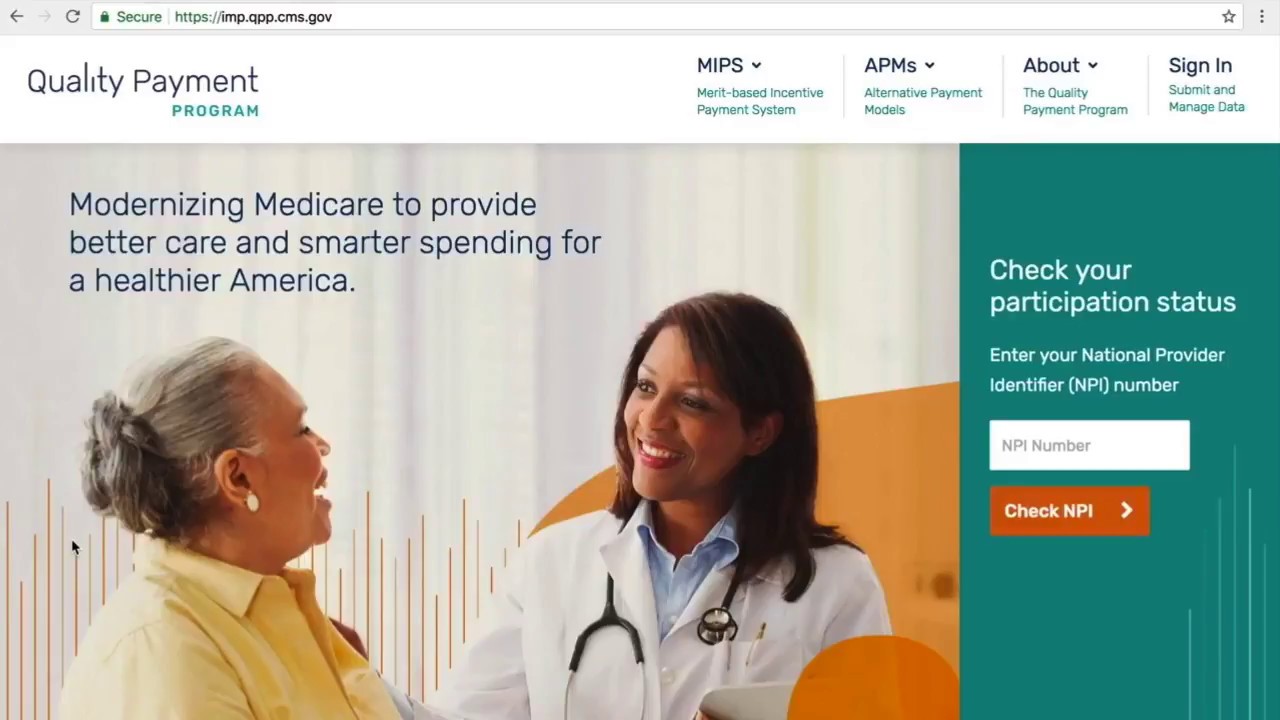This image captures a screenshot of the CMS Quality Payment Program (QPP) website. On the page, there are two women engaged in conversation. The woman on the left is a doctor, identifiable by her white coat and stethoscope. The other woman, on the right, is wearing a white shirt. Above them, a prominent text banner reads, "Modernize Medicare to provide better care and smarter spending for a healthier America."

At the top of the webpage, there is a search bar displaying the URL, app.cms.gov. Below the search bar is a navigational white band with the Quality Payment Program label, and links to MIPS (Merit-Based Incentive Payment System), Alternative Payment Models, and sections like "About the Quality Payment Program," "Sign In," and "Submit and Manage Data."

To the right of the women, a green rectangle contains instructional text: "Check your prescription status, enter your National Provider Identifier (NPI) number." Below it, there's a field to enter the NPI number and an orangey-red button labeled "Check NPI" accompanied by a small forward arrow icon.

The doctor appears to be seated on an oversized orange chair, and an orange circle is superimposed beneath and to the right of her. Additionally, thin orange lines that resemble graph lines extend from the doctor towards the other woman, creating a visually striking, albeit slightly strange, effect.